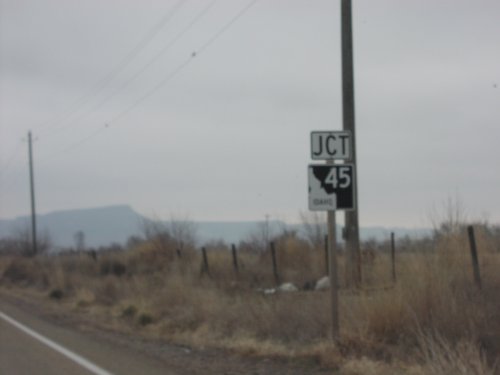The photograph depicts an outdoor, rural roadside scene in Idaho characterized by its overcast, grayish sky and mountainous backdrop. The background features a faded blue mountain range with gentle slopes extending from left to right, outlining a scenic horizon. The foreground showcases a gravel roadside bordered by a solid white line on the gray pavement. Adjacent to the road is a patch of dry, brownish-green grass interspersed with shrub brush, and crooked wooden fence posts lining a ditch. Prominently in the middle ground are two tall wooden telephone poles with power lines stretching between them. One of these poles stands near the right side of the image. Slightly to the left and in front of this pole is a thin wooden post supporting two metal signs. The top sign is a white rectangle displaying the black letters "JCT," and below it, a black square sign featuring the white outline of the state of Idaho with the number "45" inside. This cohesive description captures the scenic, serene essence of the rural Idaho landscape underscored by the overcast sky and defining infrastructural elements.